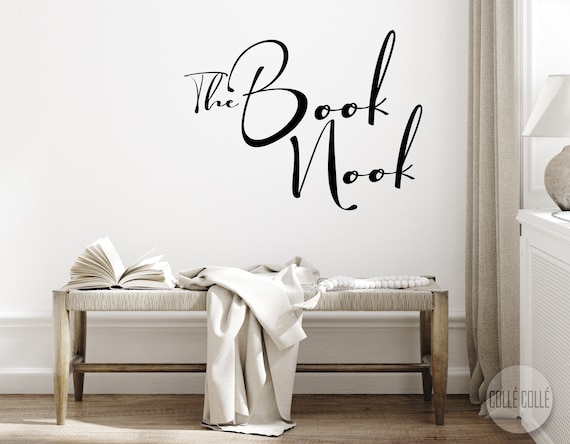In this cozy home setting, a white wall serves as the backdrop for a serene reading nook. At the center, the text "The Book Nook" is displayed in black lettering. Directly below this is a small wooden bench with intricately woven seating. Draped over the bench is a beige throw blanket, adding a touch of warmth. Resting on the left side of the bench is an open book with blank beige pages, while a white tassel garland adds a decorative touch. The medium-colored wooden floor complements the simple, yet sophisticated neutral tones in the room. To the right side, a beige curtain partially conceals a dresser topped with a beige table lamp featuring a white shade. A subtle watermark in the bottom right corner reads "Cole, Cole" within a circular emblem.